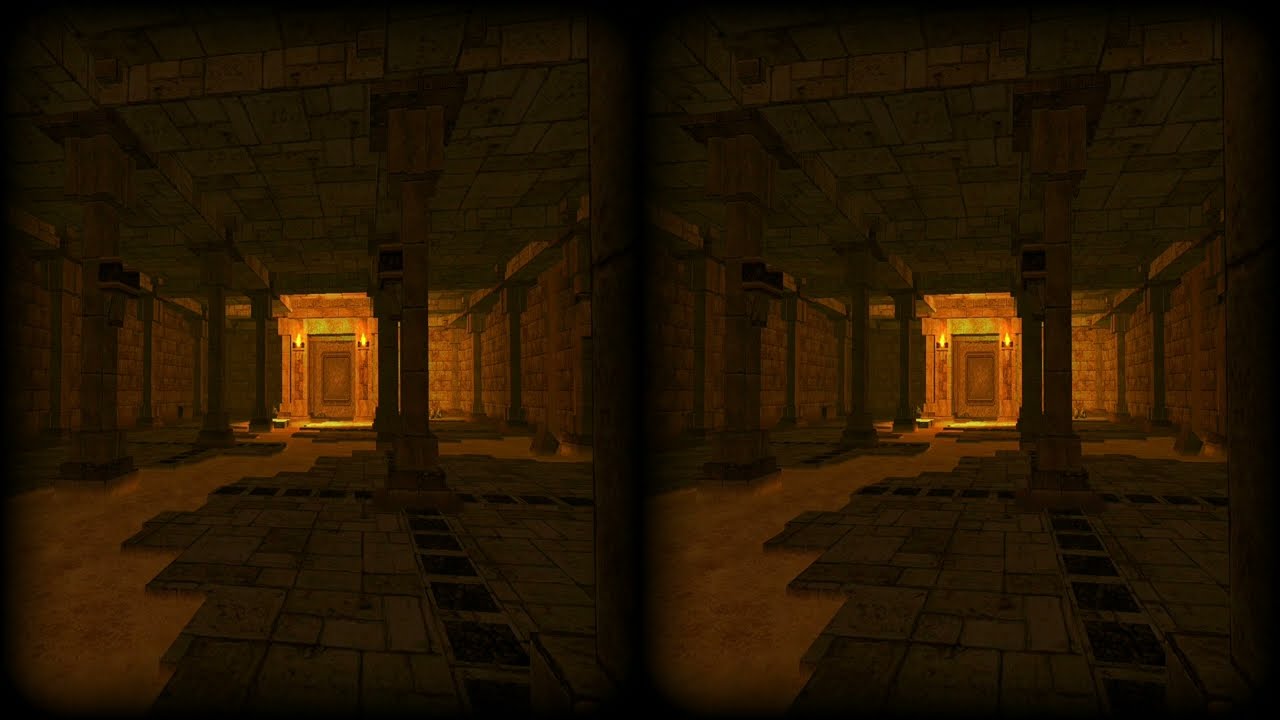The image is a side-by-side pair of what appear to be nearly identical screenshots from a video game, presented in a rectangular format measuring approximately six inches wide and three inches high. A black border with a fade effect frames the images, becoming lighter as it approaches the center vertical line that splits them. Each side depicts a slightly different perspective of the same scene, reminiscent of a view through virtual reality lenses.

The depicted scene is an ancient, archaeological temple situated in a desert environment. Sand covers parts of the stone-tiled floor, and large brown stone columns rise up, supporting the structure. The walls are constructed from large sand-colored bricks, and the ceiling is made of similar gray stone tiles. At the far end of the room, a grand stone doorway is flanked by two pillars, each adorned with a lit torch that serves as the primary source of illumination, casting an inviting, yet eerie glow on the entrance. The viewer is left with a sense of intrigue and beckoning to explore the mysterious, dimly lit temple further.